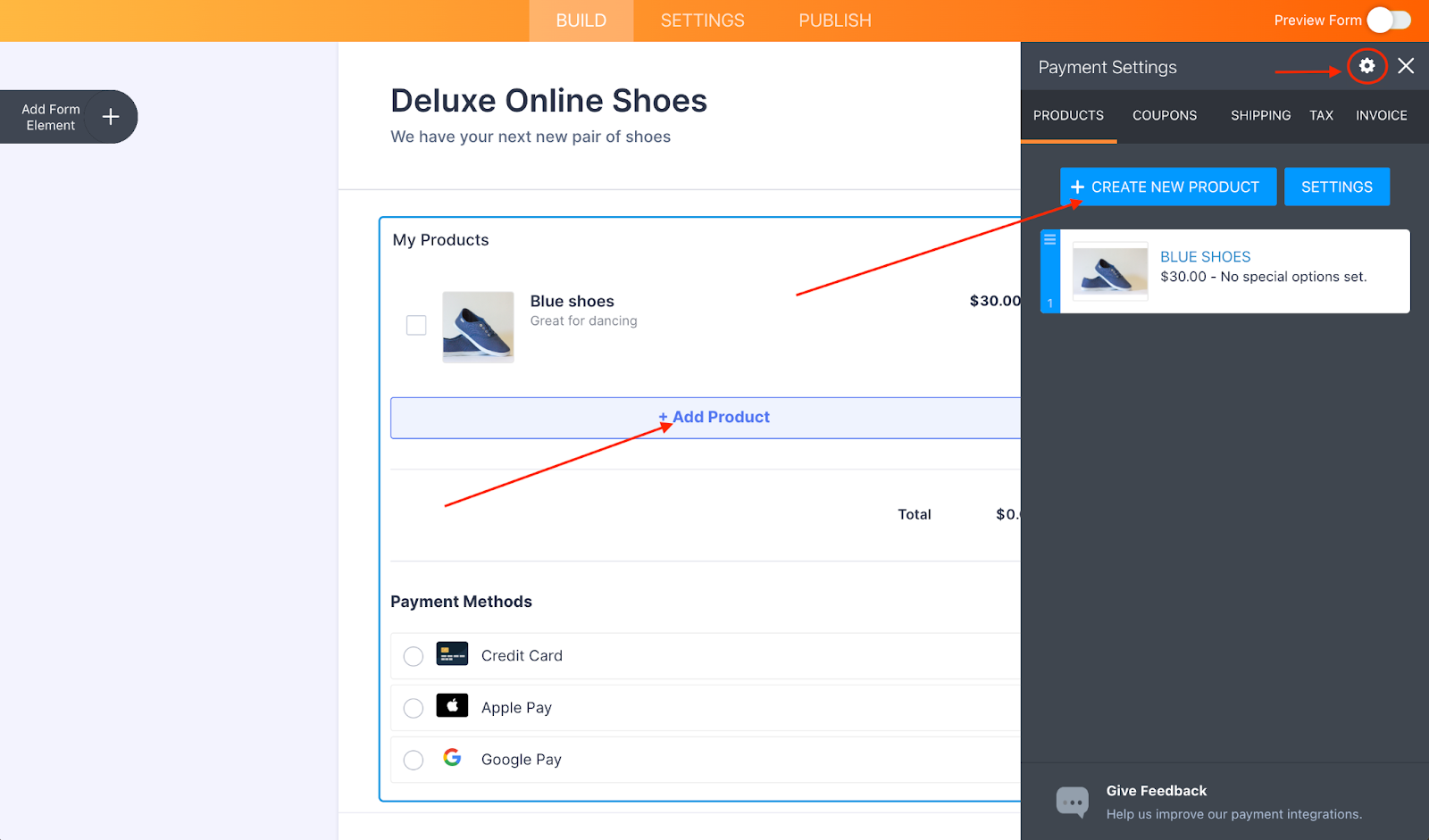Here's the cleaned and detailed caption:

---
The image displays a screenshot of a website interface. At the top, there's an orange and gold banner with white text in the center that reads "Build, Settings, Publish." In the upper right corner, there is a "Preview Form" option accompanied by a toggle switch. Below this banner, a large white rectangular section prominently features the bold text "Deluxe Online Shoes," followed by the tagline, "We have your next new pair of shoes." In this section, there’s also a square photograph of a pair of blue sneakers labeled "Blue Shoes, Great for Dancing," priced at $30. Above the photograph, in the upper left corner, the section title "My Products" is visible. Beneath the photograph, there is a light blue banner with blue text that says "Add Product," highlighted by a red arrow pointing to the word "Add." At the bottom of the screenshot, black text indicates available payment methods: Credit Card, Apple Pay, and Google Pay.

---